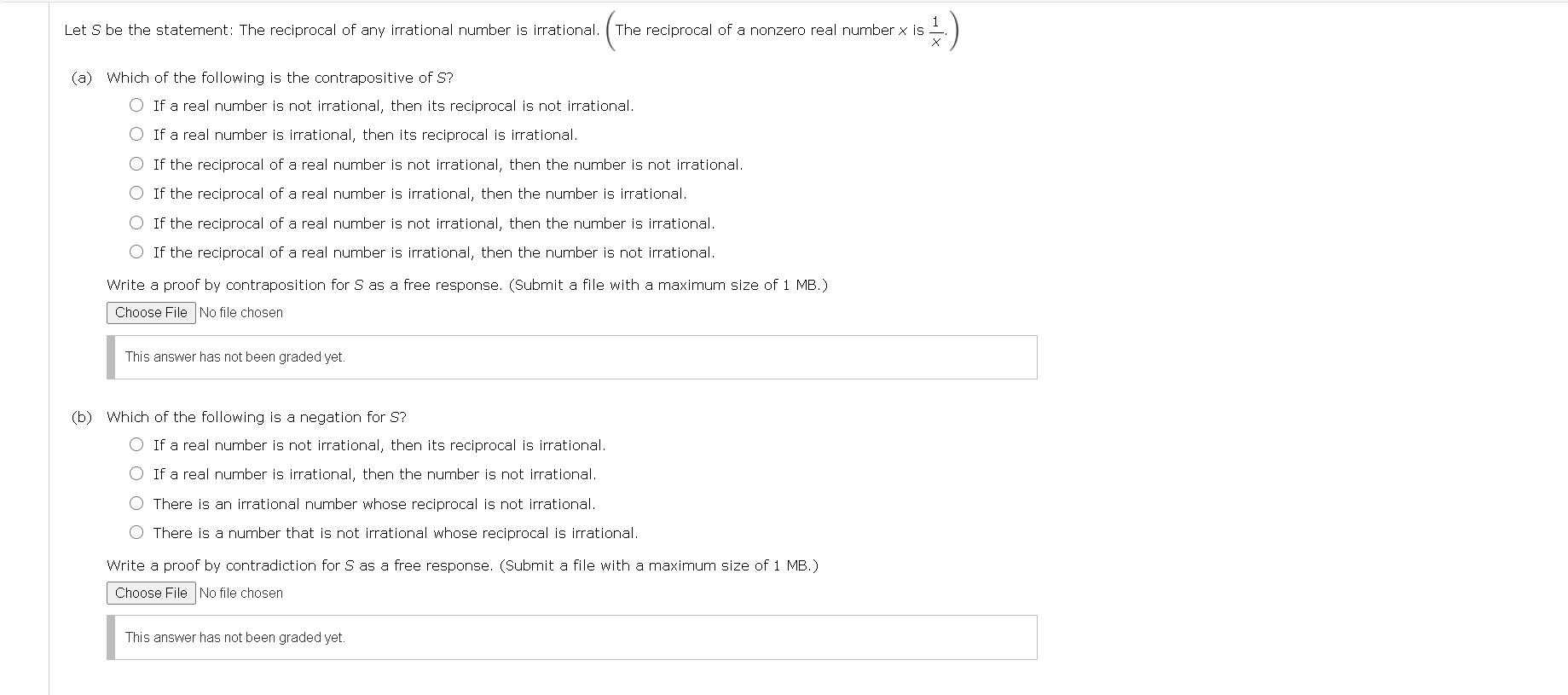Screenshot of a Test Interface Featuring Contrapositive and Negation Questions

The image is a screenshot of a digital test or survey interface, predominantly white with black text. It appears to be addressing mathematical concepts, specifically contrapositive and negation of statements. The text comprises two main questions labeled as Question A and Question B.

**Question A**: 
- Statement: **Let S be the statement "The reciprocal of any number is rational."** In parentheses, an additional clarification states, "**The reciprocal of a nonzero real number X is 1/X.**"
- The prompt under Question A asks, "**Which of the following is the contrapositive of S?**"
- Six multiple-choice options are listed to choose from.
- At the bottom of this section, there's an instruction to "**Write a proof of contrapositive for S as a free response.**" It notes to "**Submit a file with a maximum size of 1 megabyte**," followed by a "Choose File" button. To the right of this button, text indicates "**No file chosen**," signifying that no file has been uploaded.
- Beneath the button is a note stating, "**This answer has not been graded yet.**"

**Question B**: 
- Statement: **Which of the following is a negation for S?**
- Four multiple-choice options are presented for this question.
- Similarly, this section instructs to "**Write a proof of contradiction for S as a free response.**" It repeats the file submission instructions: "**Submit a file with a maximum size of one megabyte**," followed by another "Choose File" button and the text "**No file chosen.**"
- Again, a note beneath indicates, "**This answer has not been graded yet.**"

This structured layout suggests the interface is designed for a test, likely for high school or college students, focusing on logical reasoning and mathematical proofs related to reciprocals and rational numbers.